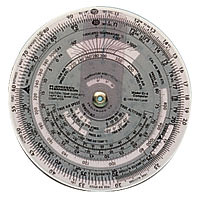This image features a small, circular device that appears to be either a scale or a compass. The device is intricately marked with numerous readings and numbers, though its precise purpose is unclear. The device has a white outer casing, while the inner section boasts a grayish hue, accented by a central screw-like element. There are grayish highlights throughout the device, complemented by scale markings and numerical indicators distributed around its circumference. Additionally, a few arrows can be observed around the device, providing further detail. The image itself is relatively small, making some of the finer text difficult to discern, and it is focused solely on this single, compact, circular device.